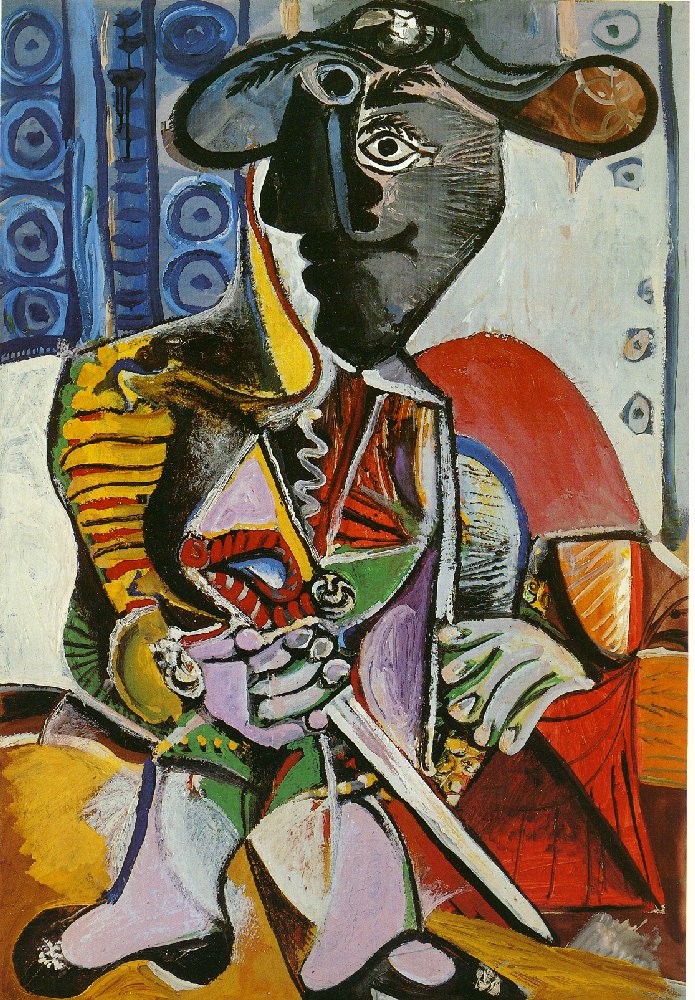This painting, titled "Matador" and done in a Picasso-esque style, features a highly abstract representation of a figure in a vividly multi-colored, elaborate outfit. The upper left corner of the image contains a blue backdrop adorned with stripes and circles, against which the character’s upper body is set. The character’s head, which is nearly two-dimensional, points to the left, showing one prominent eye and an extraordinarily large nose. The figure dons a hat reminiscent of 19th-century military attire, with hues of gray and brown.

The Matador's outfit is complex and colorful: the right sleeve is yellow with red lines, while the left sleeve is orange. The torso is clad in a strikingly varied jacket that includes shades of pink, green, and red. A red cape lined with yellow drapes from the left, revealing a vivid ensemble. The character grasps a silver sword with a red handle in one large, clumsy, cartoon-like hand, with visible fingernail beds shaded in light green and lavender. The figure’s legs, clad in green knee-length pantaloons, are grotesquely formed, wearing black low-heeled shoes with emblems, and resting on a yellow cushion-like base in the painting’s lower left corner.